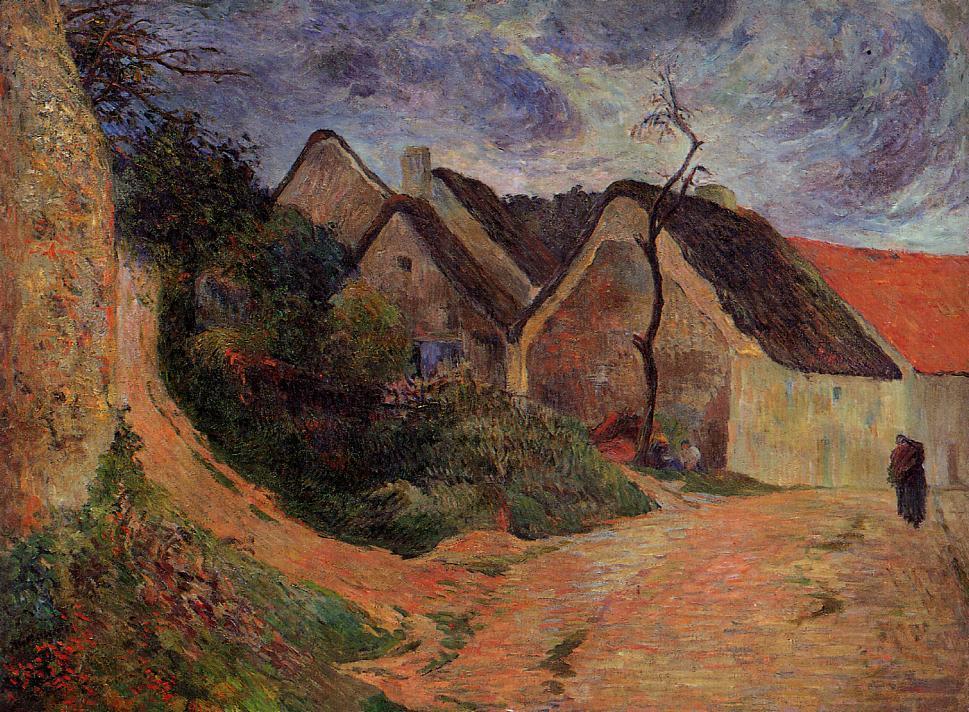This horizontally rectangular painting vividly depicts a small, rustic town set against a dramatic, stormy sky. Dominating the foreground on the right is an old building with worn stucco or concrete walls and a brown roof. A striking, tall, branchless tree rises behind it. Adjacent to this structure, another building with gray walls and a red roof stands, while a larger building is visible further along. In the scene beyond these structures, the tops of mountains pierce the horizon.

The sky is a tumultuous blend of dark and light clouds, painted in curved strokes of white, brown, and gray, giving a sense of approaching storminess. On the far left, a sheer, bare cliff ascends vertically out of view, adding to the rugged terrain. The mid-left of the painting features a large, texturally rich tree trunk with interwoven shades of brown, orange, yellow, and white, and some emerging branches. Dense greenery, with touches of red, covers the ground in front of the buildings.

People animate this tranquil village scene: one person is noticeable, sitting in front of a home, while another figure can be seen standing outside a house on the right, dressed entirely in brown. The ground beneath them is a patchwork of dirt, grass, and autumnal hues of brown and red. Despite the sky's ominous appearance, the overall setting is bright and suggests daylight, further enriched by the vivid, harmonious use of color.